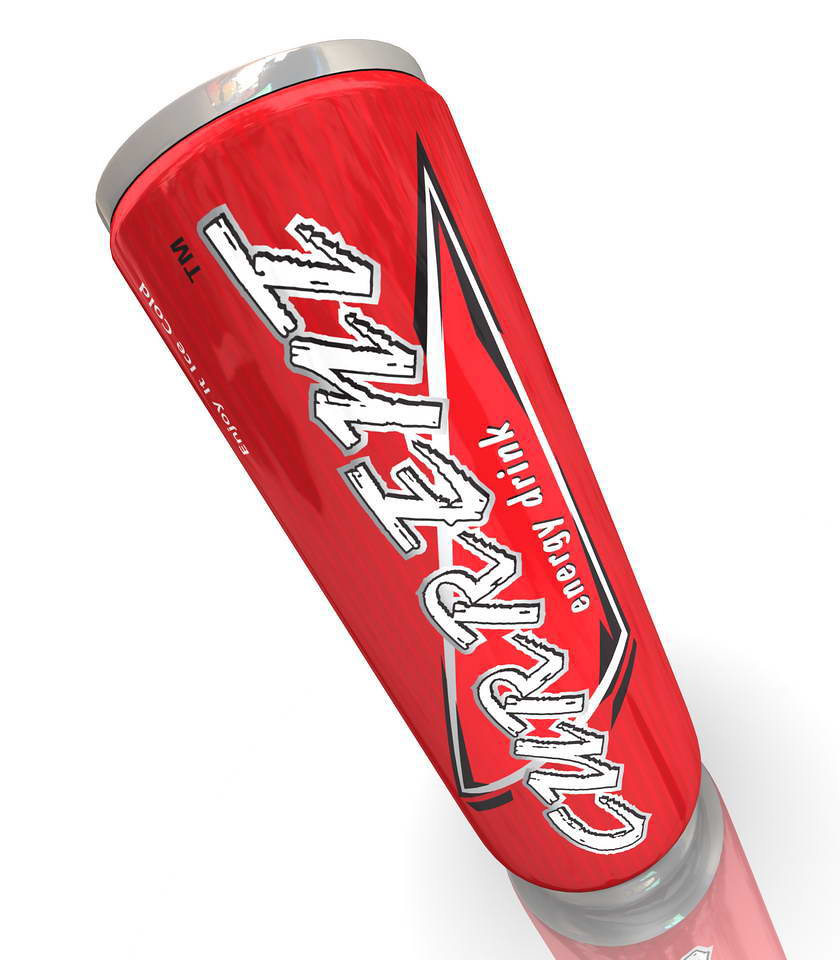In the center of the image, there is a sleek, red-colored energy drink can. The can is set against a minimalistic, pure white background, which draws full attention to its vibrant hue and branding. Dominating the label in bold, white lettering, the word "CURRENT" is prominently displayed, each letter clearly printed as C-U-R-R-E-N-T. Beneath this, the label reads "ENERGY DRINK," also in white text. On the top left corner of the can, the letters "T-M" are subtly printed. The can casts a faint reflection or shadow on the bottom right side of the white surface, adding depth to the otherwise stark and simple composition.